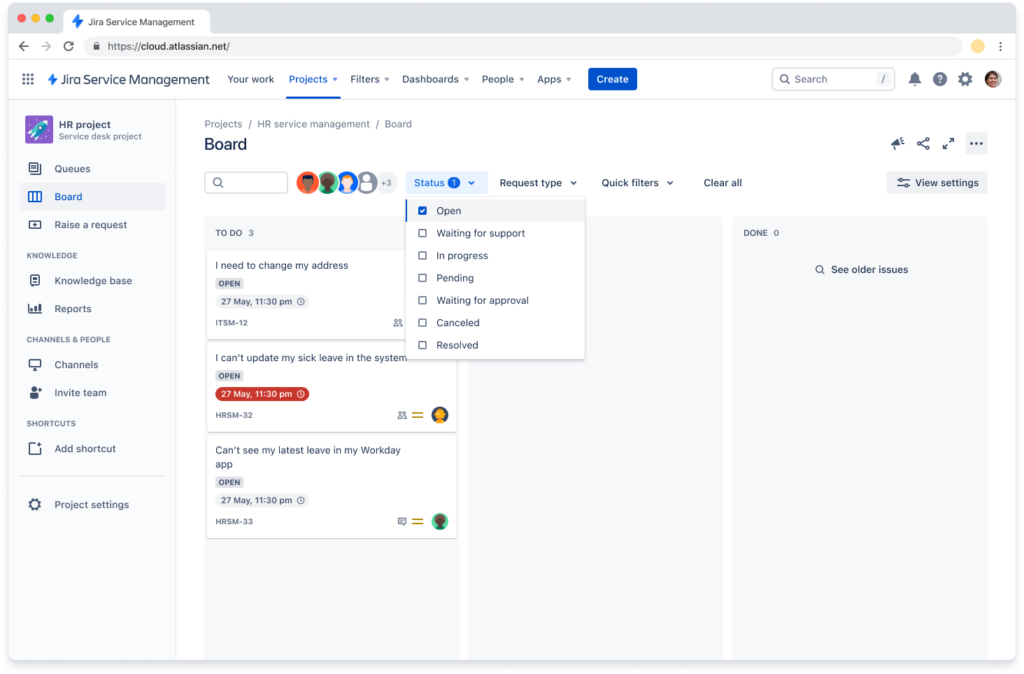The image displays a Chrome web browser open to a JIRA Service Management page, characterized by its white background and gray top bar. In the top menu, options include “Your Work,” “Projects” (currently selected), “Filters,” “Dashboards,” “People,” “Apps,” and “Create.” A search bar is also present. 

On the left, there are sidebar items listed: “HR Project,” “Service Desk Project,” followed by menu options such as “Queues,” “Board,” “Raise Request,” “Knowledge Base,” “Reports,” “Channels,” “Invite Team,” “Shortcuts,” “Add Shortcut,” and the final item, “Project Settings.”

The main content area displays the Project Board under “Projects / HR Service Management / Board.” The board resembles a virtual whiteboard featuring various notes labeled under different sections. One section, marked “To View,” includes notes stating, “I need to change my address,” “can’t update my sick leave in the system,” and “can’t see my latest leave in my Workday app.” Additionally, there is a status menu for changing the status of tasks, and a “Done” section along with options for “View Settings” and “Filters.”